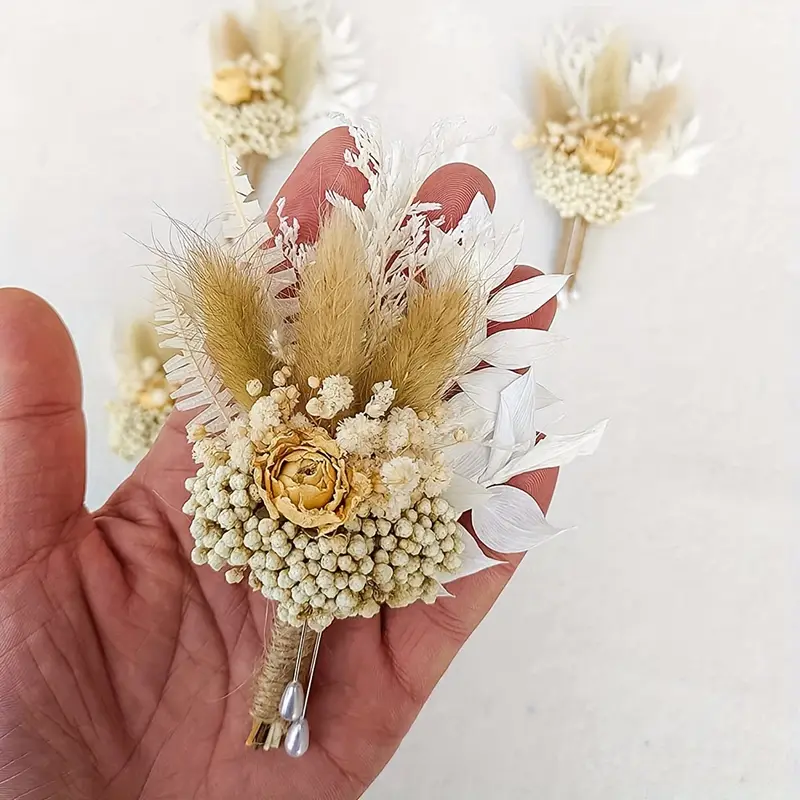The image is a color photograph in a square format, showcasing a hand-fashioned boutonniere made from natural materials. The boutonniere is held in the palm of a person's left hand, which extends from the bottom left corner of the image with the thumb on the left side and the upturned palm toward the center. In the center of the palm sits the boutonniere, featuring a central ivory rose surrounded by white baby's breath and miniature feathery sprigs of gold-colored grass. 

The boutonniere is secured with light-colored twine, and two hat pins with pearl heads are positioned near the stem, ready to attach to a lapel. The back part of the boutonniere is adorned with white foliage that includes fern-like leaves and grass. In the background, a light gray surface displays two additional boutonnieres that are slightly out of focus. The style of the photograph is a representational realism, capturing the intricate details and natural textures of the boutonnieres in a product photography setting.